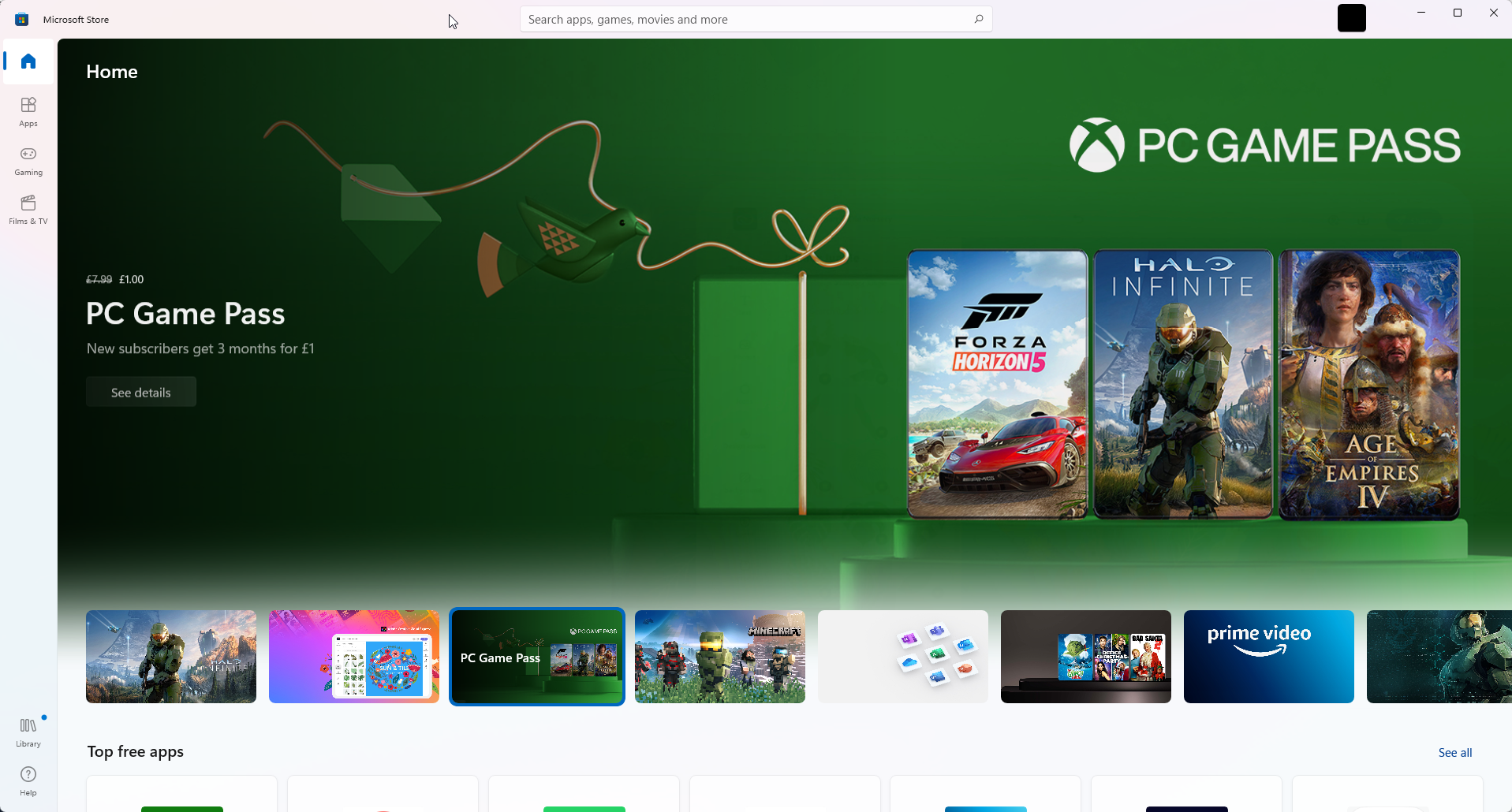The image depicts a website interface with a prominent light faded pink banner at the top, which extends down the left side before transitioning into blue. At the center top of the page, the "Microsoft Store" logo is displayed alongside a shopping bag icon. Near the top right, a mouse arrow pointer hovers close to the search bar, which contains placeholder text, "Search apps, games, movies, and more," accompanied by a magnifying glass icon.

To the right of the search bar, there is a black square containing three symbols: a minimize line, a full-screen box, and a close "X" button. The left sidebar features menu options on a white background, starting with a blue-highlighted 'Home' button, followed by 'Apps', 'Gaming', 'Films & TV'. 

The main content area of the site is framed by this border, with a dark blue or very dark green gradient on the left side that fades into a light green gradient on the right. Dominating this section is the "PC Game Pass" title in bold, white capital letters. Below this, a promotional text announces, "PC Game Pass, £1 for the first month. New subscribers get three months for £1. See details."

In the center of the page, a present graphic is displayed, flanked by three game thumbnails. At the bottom of the image, although partially cut off, there are several icons spread out beneath the heading "Top Free Apps."